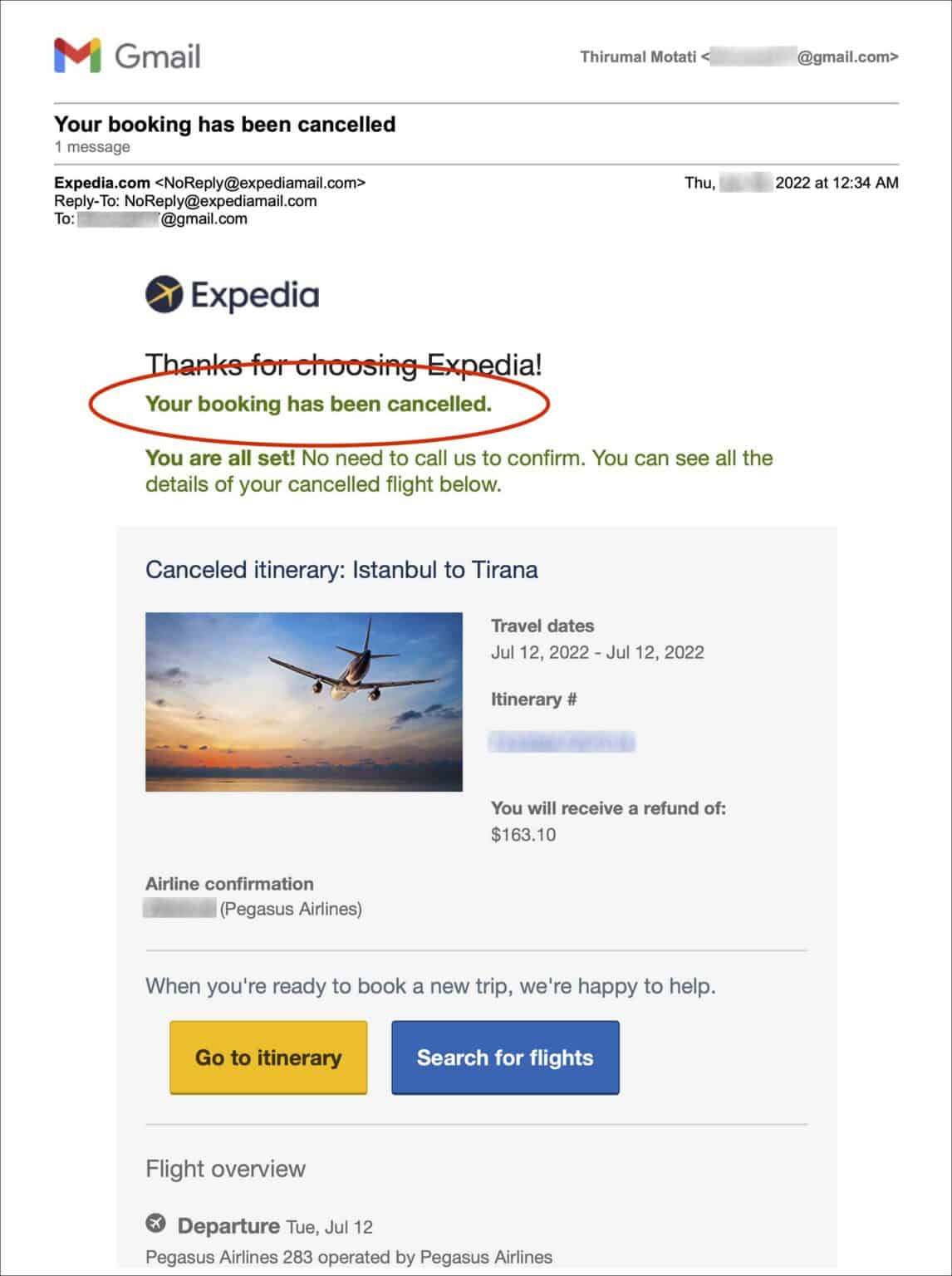The image showcases a screenshot of an email displayed on a white background with a light black border. In the upper left corner is a brightly colored "M" icon, indicating the Gmail logo. To its right, an email address is present but blurred for privacy. Below the address is a horizontal line. 

Underneath the line, the text "Your booking has been cancelled" is prominently displayed, with "1 message" indicated next to it. Further down another horizontal line appears. Beneath this line is the information from the email sender: "Expedia.com," "no-reply@expediamail.com," with a date blurred out, and a timestamp reading "2022 at 12:34 AM." The email is addressed to a Gmail address which is also blurred out. 

The main body of the email starts with a header "Expedia," followed by "Thanks for choosing Expedia." The primary message, which reads "Your booking has been cancelled," is circled in red for emphasis.

Below the circled text, it states, "You're all set, no need to call us to confirm. You can see all the details of your cancelled flight below." At the bottom of the screenshot, there is a gray box labeled "Cancelled Itinerary" with details of the flight route from Istanbul to Tirana.